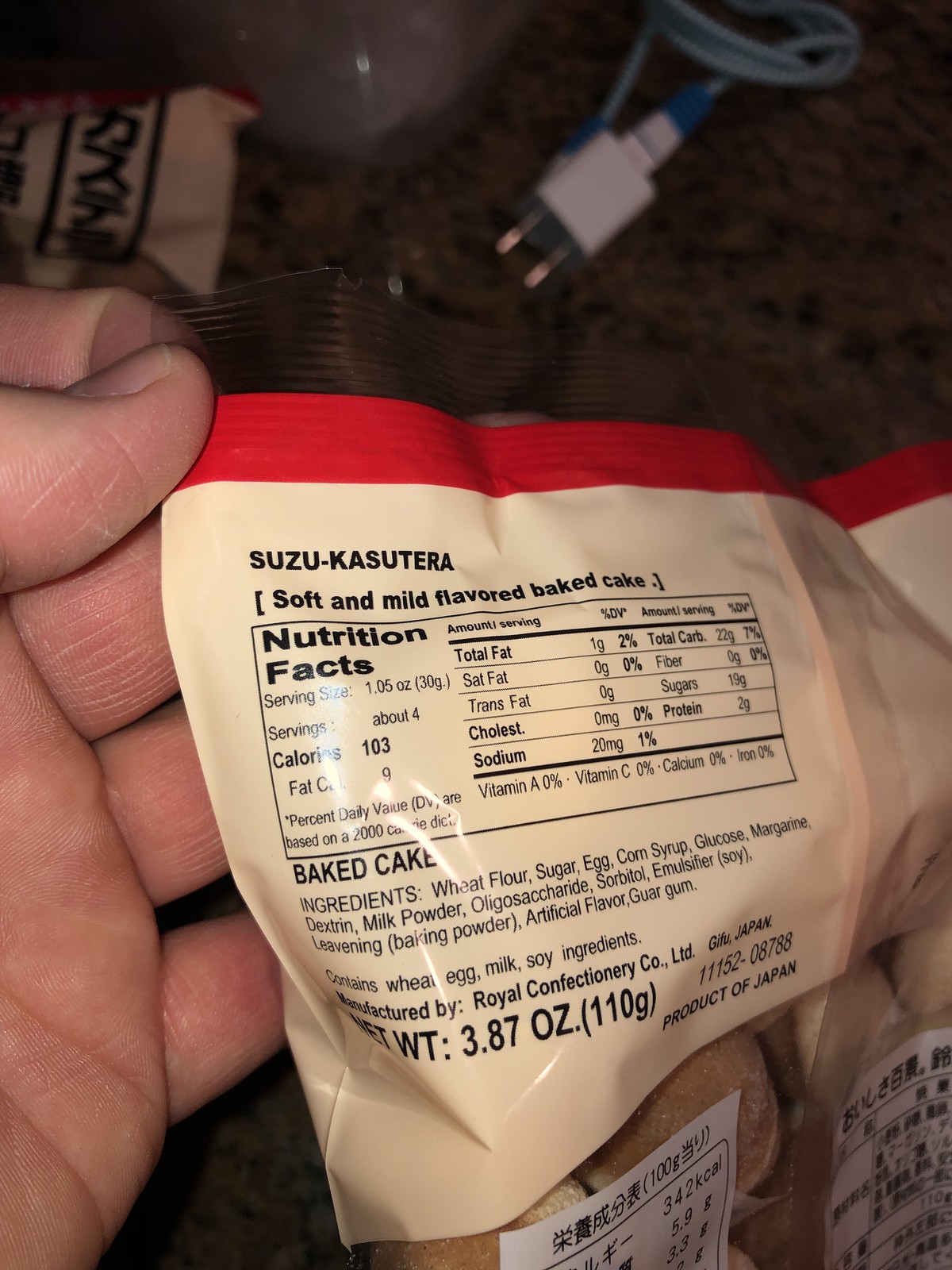In this image, a person, identifiable by their Caucasian hand, is holding an unopened package of Suzu Casutera, a brand known for its soft and mild-flavored baked cakes. The packaging of the product is a subtle light peach color, accentuated by a vibrant red strip at the top, giving it a classic, eye-catching appeal. The reverse side of the package is visible, prominently displaying the nutrition facts. It indicates that each serving of the cakes contains 103 calories, with 1 gram of total fat comprising 2% of the daily recommended intake. The list of ingredients includes wheat flour, sugar, eggs, corn syrup, glucose, and milk powder, highlighting the simple, wholesome components used in the making of these delightful treats.